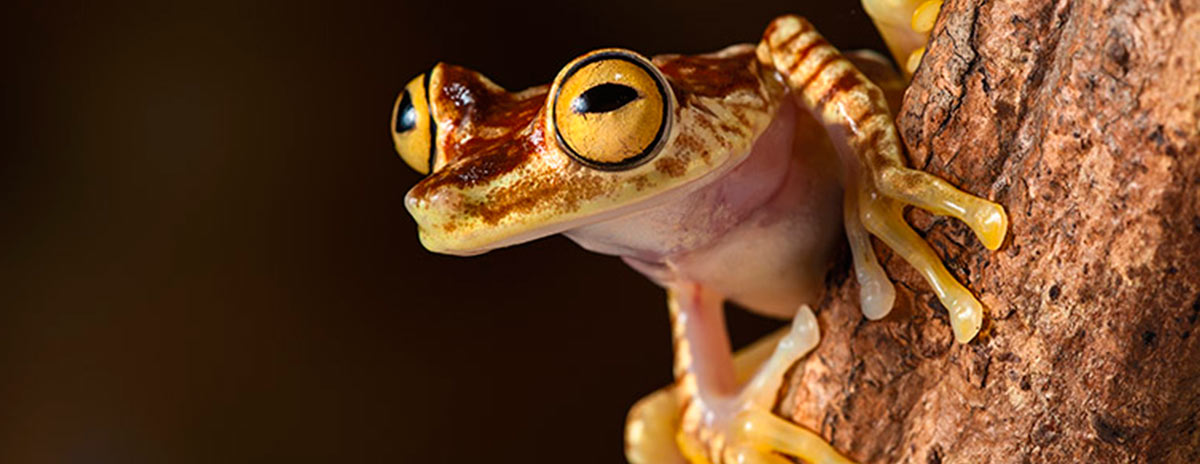This wildlife image features a close-up, panoramic view of a tree frog centrally positioned on a rough-textured, brown tree branch. The tree frog displays a palette of yellow and brown hues with rust-colored stripes adorning its body. Its head is marked with brown blotches, and it is characterized by two prominent, bulbous, yellow eyes with thin black, horizontal pupils. The frog's underbelly is primarily white with a slight pink tint. It appears to be smiling and has a sticky appearance. The tree frog is gripping the branch with its three-fingered front feet positioned on top and its lower feet placed behind it, propping itself up vertically. The left side of the image is pitch black, providing a stark contrast to the vivid details of the frog and tree branch.